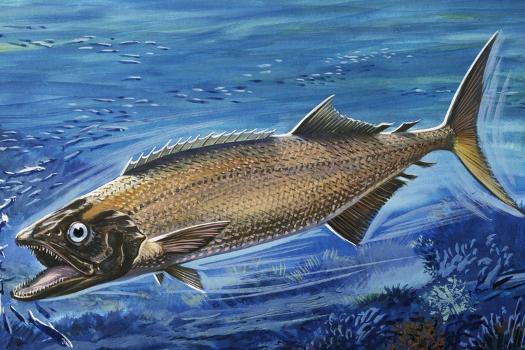This vibrant painting captures an underwater scene featuring a large predator fish actively hunting. Dominating the center of the image is a side-profile of a long, light brownish fish with an open mouth lined with tiny, jagged teeth. Its distinct darkish face and prominent white eye with a black speck add to its predatory appearance. The fish's body showcases a variety of colors including white, pink, dark brown, green, and tan with fins positioned on the top, bottom, and back, extending to a tail that curves slightly upwards. Surrounding the fish are several smaller, grayish minnows creating ripples in the blue water. The background showcases a rich blue hue simulating the ocean, with some hints of movement and waviness. In the lower right corner, vibrant coral and underwater plants—colored in shades of brown, green, and bluish-green—add depth and context to the scene, enhancing the aquatic environment depicted in this detailed and colorful underwater tableau.